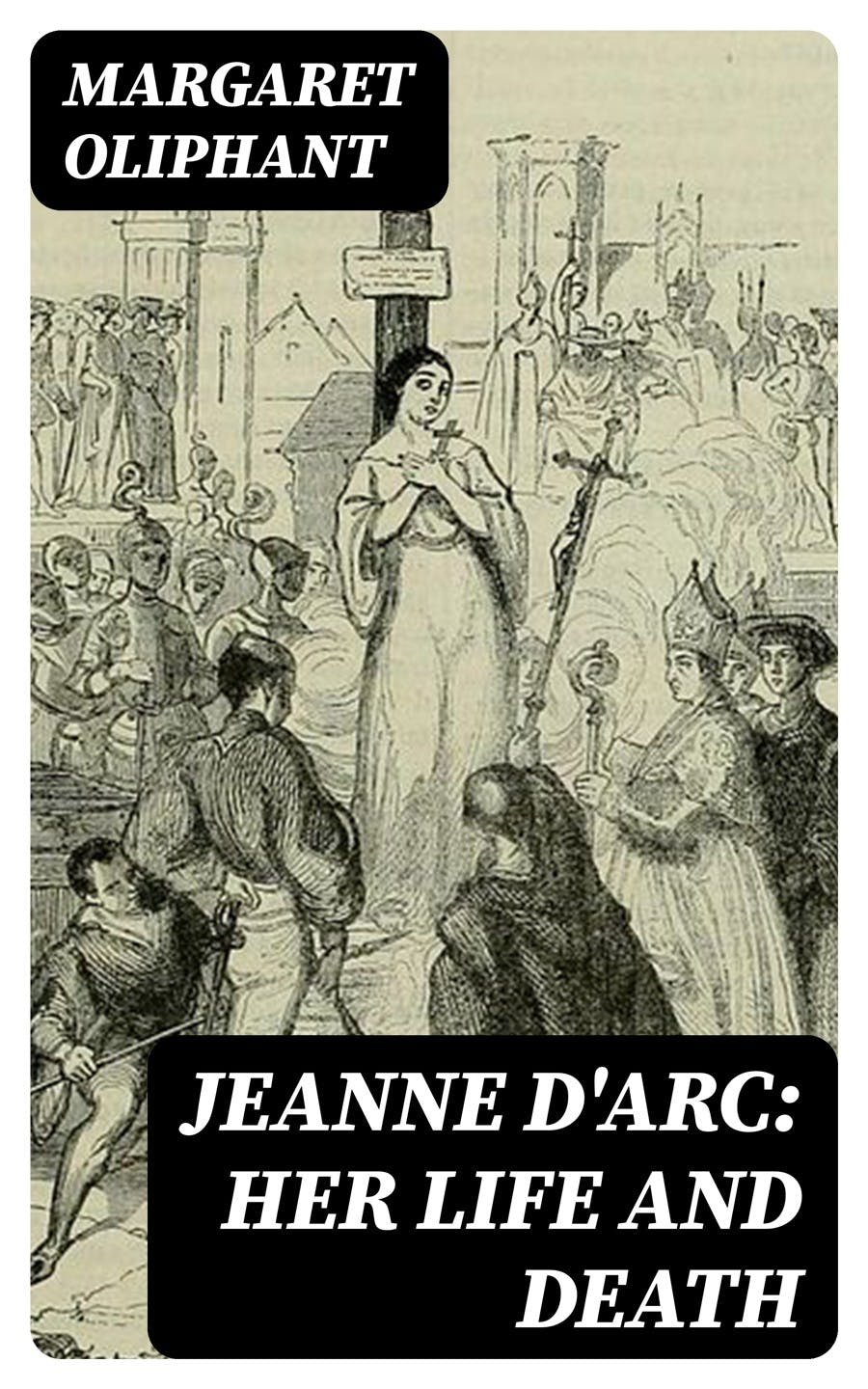The cover of the book, titled "Joan of Arc, Her Life and Death" by Margaret Oliphant, features a detailed black-and-white illustration of Joan of Arc. Joan, depicted as a young woman in a long gown, is bound to a large wooden stake, indicating the moments before her execution by fire. A faint smoke rises, hinting at the fire starting behind her. She clutches a cross, signifying her faith. Surrounding her is a tumultuous crowd, including clergy, knights, and men-at-arms, with detailed depictions of crosses and churches among the background elements. The author's name, Margaret Oliphant, is prominently displayed in a black box with white lettering at the top left. Another black box with white lettering at the bottom right states the book's title.